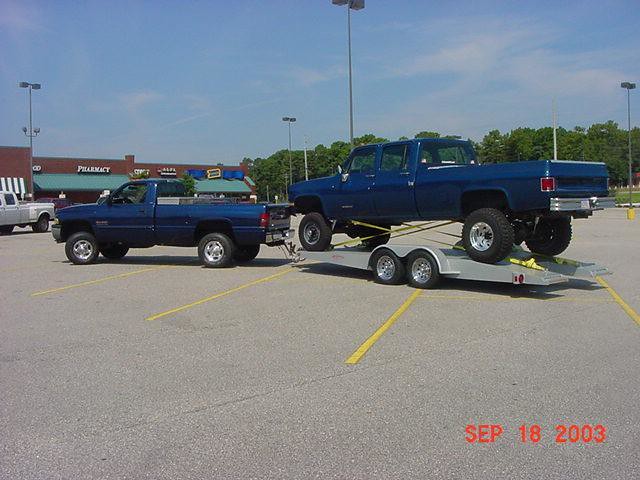This image, captured on September 18, 2003, depicts a clear day in a parking lot beneath a vivid blue sky with scattered white clouds. The parking lot itself features faded blacktop with distinctly painted yellow lines demarcating the parking spaces. Dominating the scene is a blue pickup truck parked askew across the yellow lines, towing a silver trailer. This trailer carries an older, larger blue pickup truck with four doors, a taller profile, larger wheels, and an extended pickup bed. In the background, there's a strip mall with a red brick facade, where one store's sign reads "Pharmacy" and another store with a blue awning features a yellow sign. Further back, tall lights designed to illuminate the lot are visible, alongside lush green foliage that hints at a nearby forest or park. Adding depth to the scene, a small portion of a gray truck is slightly visible entering from the left side of the frame.